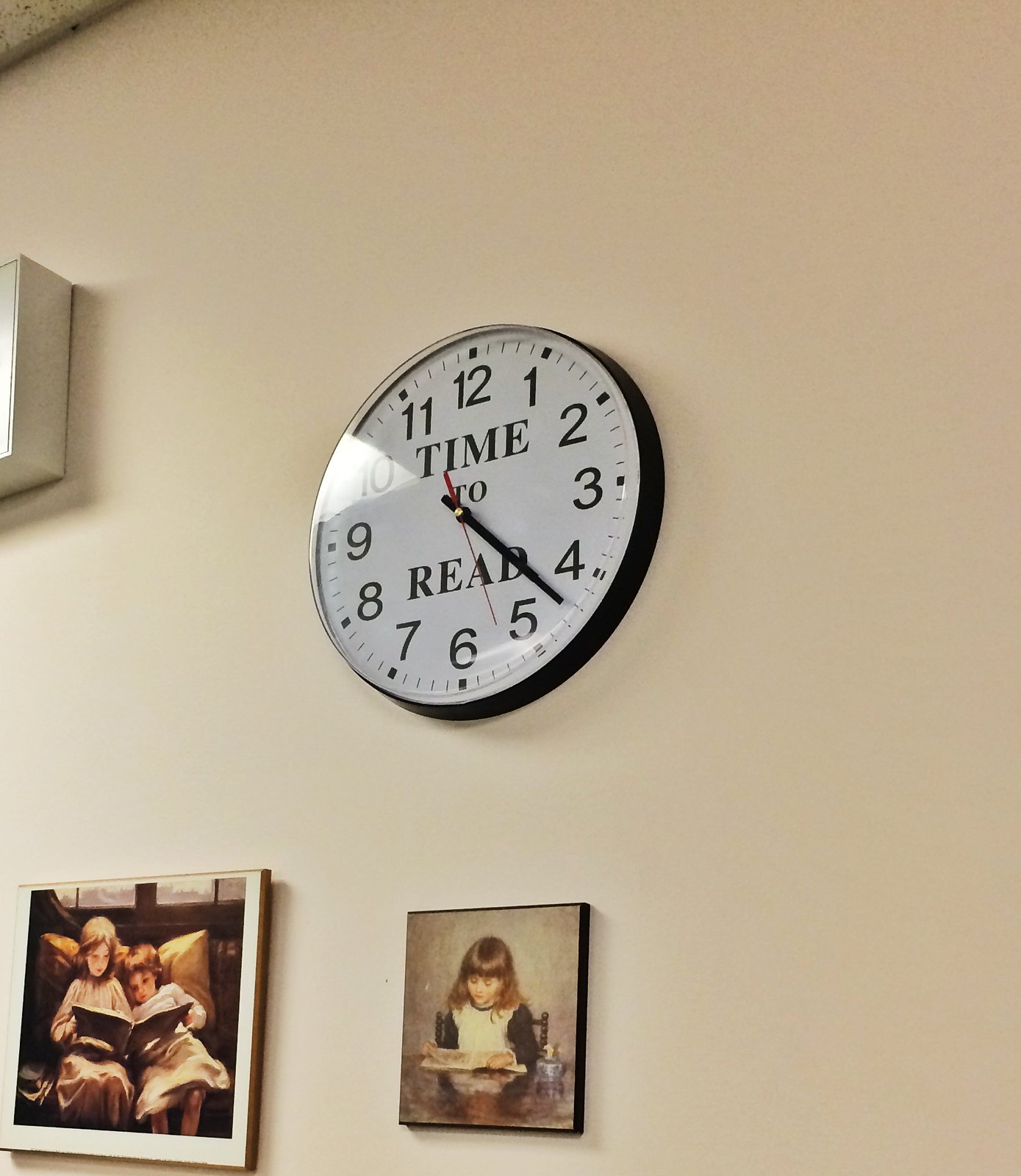The image features a beige wall adorned with a clock prominently displaying the phrase "Time to Read" on its white face. The clock has black hour and minute hands, a red second hand, and black numerals encircling its edge. Below the clock, there is a vintage photograph of a young girl. She wears a pinafore over a blouse and is engrossed in reading a book; her long brown hair cascading around her shoulders. Beside her, two children are seated on a couch, side by side, sharing and reading a book together. Mounted on the wall is a shiny, boxy object whose exact nature is indeterminate—it could be a cabinet or a picture. Above, part of a drop-down white ceiling is visible, adding to the cozy, nostalgic ambiance of the scene.